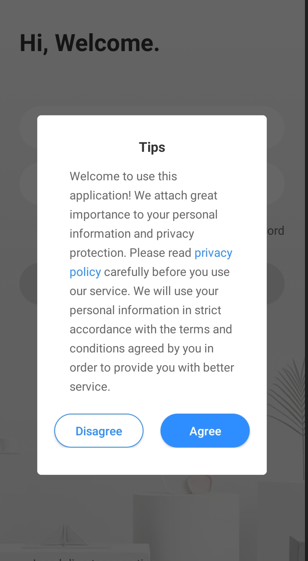The screenshot features a user interface with a very dark gray background. In the upper left corner, bold black text reads "Hi. Welcome." Below this greeting is a vertically elongated white rectangular box. Centered at the top of this box, "Tips" is written in bold black text. Further down within the box, light gray text states: "Welcome to use this application. We attach great importance to your personal information and privacy protection." Following this statement, the words "privacy policy" appear in blue text. The message continues in gray text: "Carefully, before you use our service, we will use your personal information in strict accordance with the terms and conditions agreed by you in order to provide you with better service." At the bottom of the box, two options, "Disagree" and "Agree," are presented to the user.